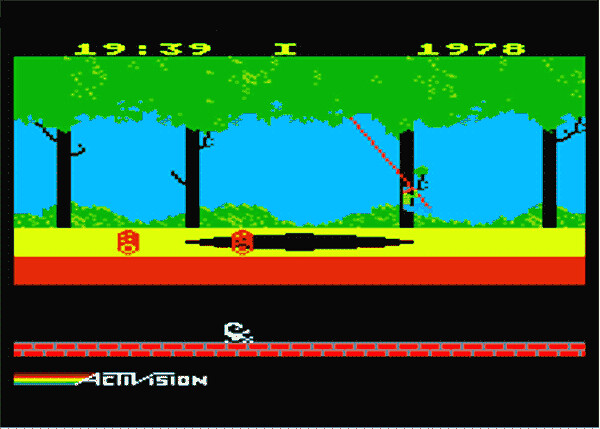The image is a screen capture from the classic video game Pitfall, featuring a distinctly pixelated aesthetic. Dominating the top of the screen is bright green text displaying "19:39" on the left, the letter "I" in the center, and "1978" on the right, all against a black background. The main art, set within a black border, depicts a forest landscape with black tree trunks and green foliage. In this scene, a small character dressed in a green top and blue pants, swinging from a red rope over a black pit, can be seen. Below this, yellow ground with red obstacles or logs is visible, while an underground area is indicated by a red brick path with a white pixel art scorpion present near the bottom center of the screen. At the bottom left of the screen, the Activision logo is displayed in white text, accentuated by adjacent colored stripes in red, yellow, and green.